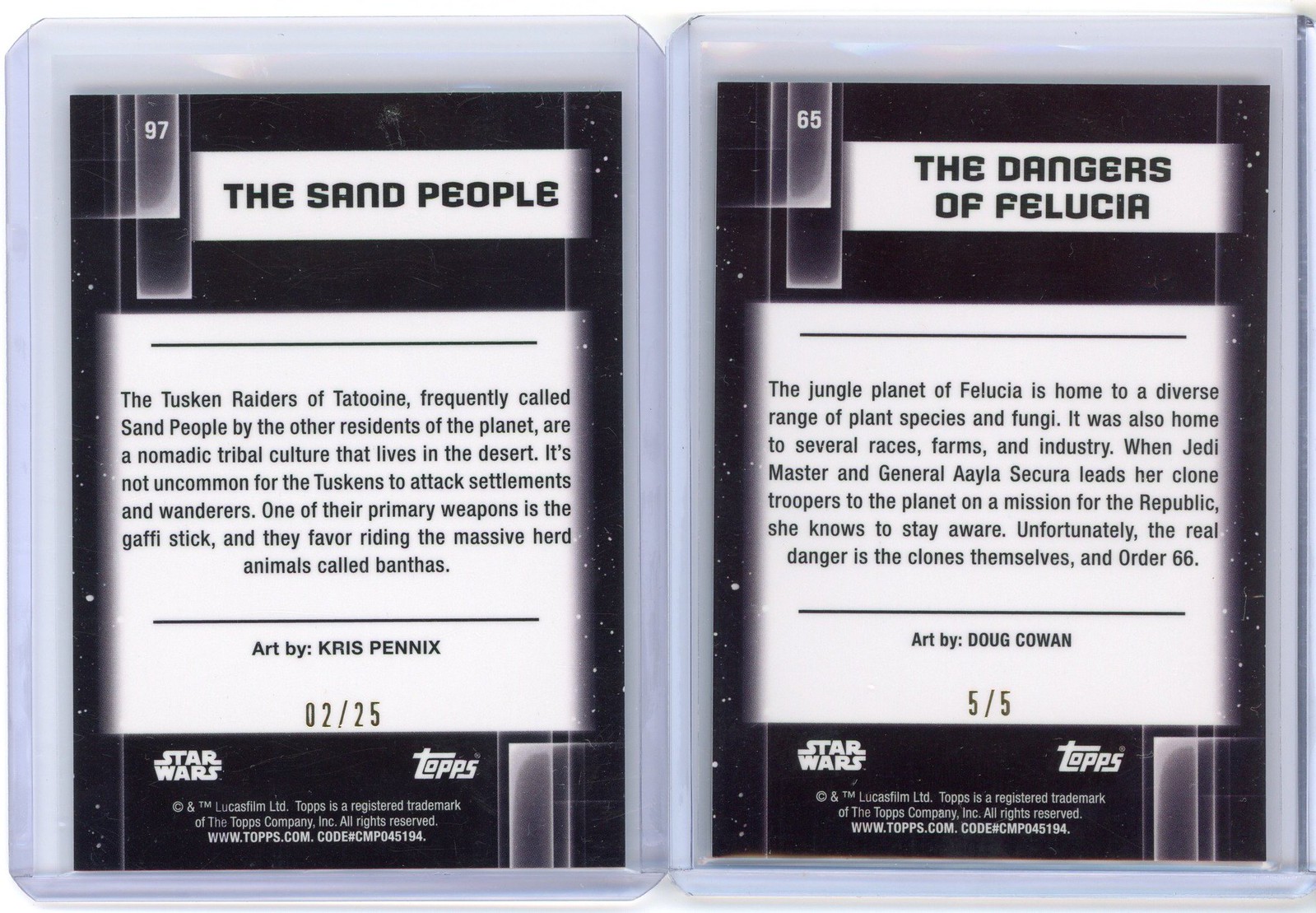This image showcases two Star Wars trading cards side-by-side, each inside a white plastic case. Both cards feature a black background with white rectangular headings and central text blocks. The card on the left, numbered 97, is titled "The Sand People." It includes a detailed description that reads: "The Tuscan Raiders of Tatooine, frequently called Sand People by the other residents of the planet, are a nomadic tribal culture that lives in the desert. It's not uncommon for the Tuscans to attack settlements and wanderers. One of their primary weapons is the gaffey stick, and they favor riding the massive herd animals called banthas." The card also cites "Art by Chris Penix, 02-25" and features logos for Star Wars, T.O.P.S., and copyright information for Lucasfilm Ltd. and The T.O.P.S. Company.

The card on the right is numbered 65 and titled "The Dangers of Felucia." Its text block reads: "The jungle planet of Felucia is home to a diverse range of plant species and fungi. It was also home to several races, farms, and industry. When Jedi Master and General Ayla Secura leads her clone troopers to the planet on a mission for the Republic, she knows to stay aware. Unfortunately, the real danger is the clones themselves in Order 66." This card also credits "Art by Doug Cowan, 05-05" and displays logos for Star Wars, T.O.P.S., along with copyright information for Lucasfilm Ltd. and The T.O.P.S. Company.